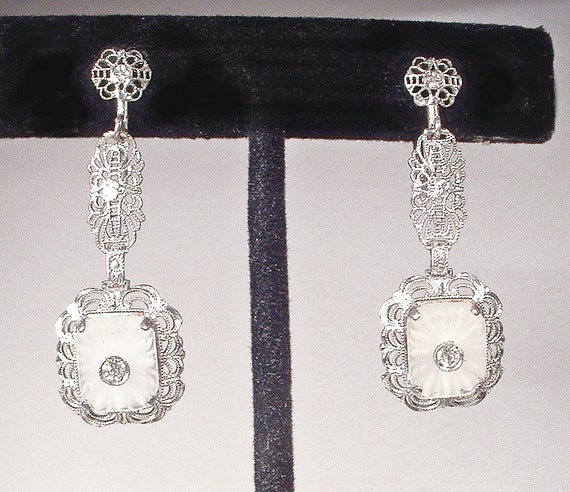The image depicts a pair of long, intricately designed silver earrings set against a soft gray background. These earrings are elegantly displayed on a holder with a thin black stem, likely made of plastic or metal, extending upwards to a rectangular top. The holder's top, possibly covered in a velvet-like material, features holes to accommodate the earrings. Each earring is adorned with a brocade pattern at the base, which advances into a larger and more elaborate brocade design. The centerpiece of each earring is a prominent rectangular white stone, encircled by intricate silver loops and swirls, adding a premium touch. These dangly earrings, likely of a push pin style, extend nearly to the shoulders when worn, showcasing their substantial length and beautiful craftsmanship.